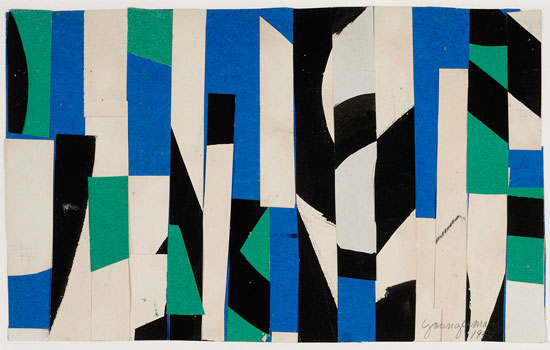The image is an abstract artwork, possibly resembling paper mache or collage, creating a mosaic-like pattern. It features a random arrangement of straight and curved lines made up of layered pieces of paper. Dominant colors in the artwork include dark blue, dark green, white, and black. These colors form long vertical stripes of varying widths, interspersed with squares and triangles of different sizes, creating a complex interplay of negative and positive space. Pencil marks are visible across the white sections, adding subtle texture. In the lower right-hand corner, the artist's signature and part of a year, 19XX, are faintly discernible in light grey. The piece appears to be mounted and may have a border, adding to its presentation.